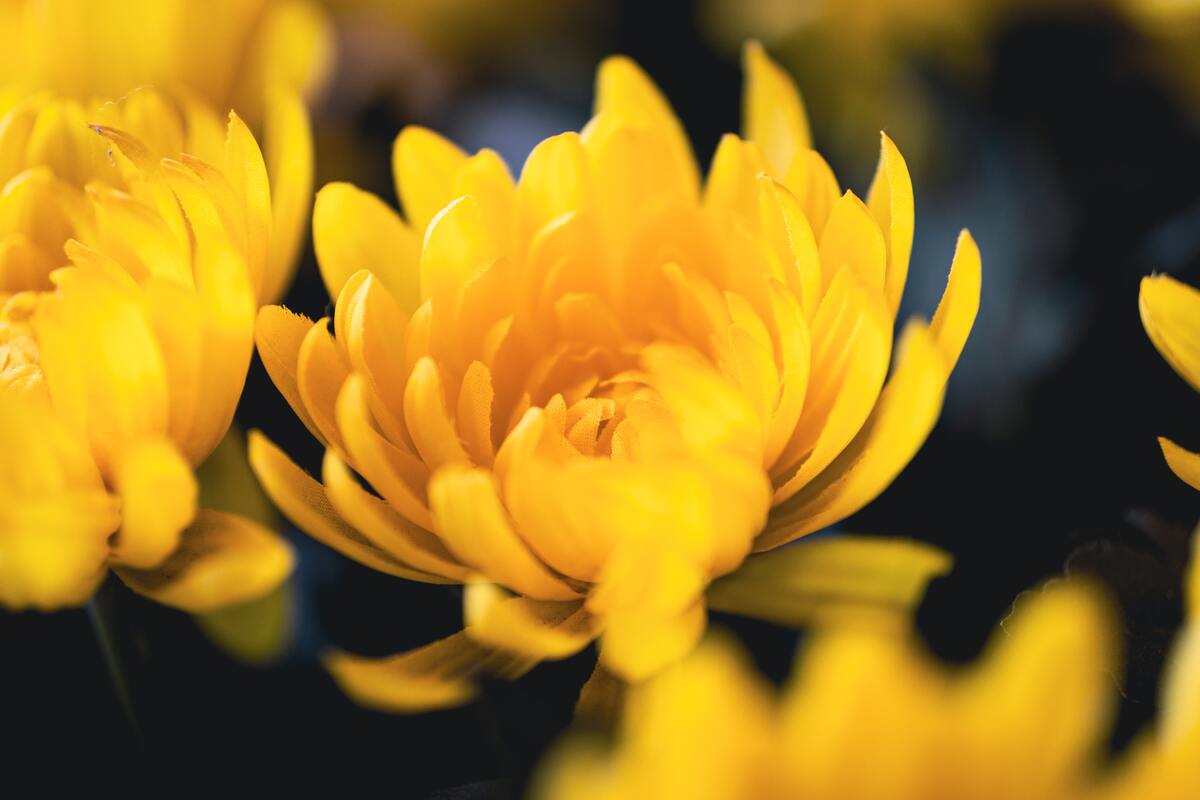The image is a high-quality, macro shot of a group of yellow flowers, with emphasis on a fully-bloomed one at the center. This central flower displays bright yellow petals that spread out from a dense core, resembling a basket or shell. Just beside it, another flower is mostly in sharp focus, revealing its side profile. The foreground features a partially visible, blurred yellow flower, while the background includes at least one more yellow flower in an even blurrier state, all set against a dark green backdrop with hints of black and light blue. The flowers have long, arching petals that converge closely together, giving a soft and vibrant appearance.